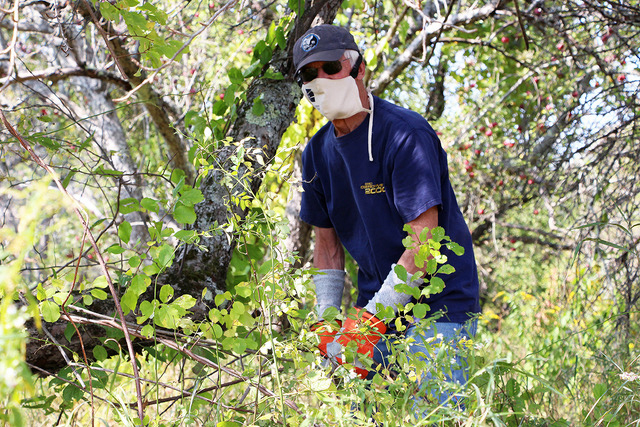The image depicts a Caucasian man in a dense wooded area, likely engaged in some form of landscaping or clearing brush. He wears a white mask, black sunglasses, and a dark navy ball cap that partially covers his white hair. His attire includes a navy blue short-sleeve t-shirt with indecipherable yellow wording, blue jeans, and white and orange gloves that extend up to his elbows. The man stands amidst tall grasses that reach up to his thighs and is surrounded by dense foliage. Notably, the scene has varied vegetation, including trees with small pink flowers in the background and others with tiny yellow flowers or red berries. The sunny day highlights the vibrant green leaves around him as he looks towards the camera, appearing to focus on his task at hand.